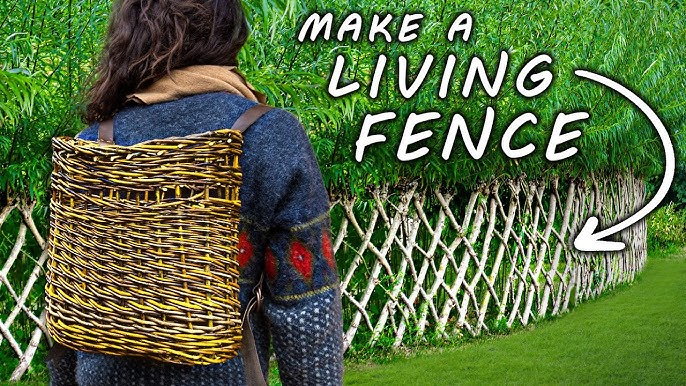In the image, a woman with long, dark hair, wearing a navy blue sweater and a tan hoodie, is prominently featured on the left side, her back turned towards the camera. She is carrying a unique backpack made of woven wooden sticks. The lush background showcases a green landscape with various trees, shrubs, and grass. At the top center, white text with a black border says, "Make a Living Fence," accompanied by an arrow pointing to a distinctive fence crafted from interwoven tree branches. The fence, which encircles a garden area, harmonizes with the natural greenery, creating an earthy and serene atmosphere. Touches of colors like green, red, blue, black, brown, dark red, yellow, and darker navy blue add to the image’s vivid palette.